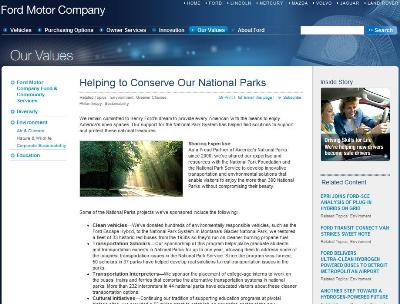This webpage screenshot features a dynamic layout with distinct sections and an engaging design. At the top, there is a prominent horizontal banner that transitions from black on the left to light blue on the right. Positioned in the upper left-hand corner of this banner, the text "Ford Motor Company" is displayed in bold white font. Running across the top edge, a horizontal menu is arranged with white text, providing easy navigation options.

Directly below this primary menu, a secondary menu continues with additional options also in white text. Situated on the far right end of this line, there is a white rectangle housing a blue search button, clearly labeled “Search” in white text.

Three lines down on the left side of the page, the heading "Our Values" appears in a light gray color. The main content area is predominantly white, occupying the left three-quarters of the screen, while a narrower gray rectangle occupies the right-hand side.

Inside this primary white segment, a prominent heading "Helping to Conserve Our National Parks" draws attention to a featured article. This section includes a brief introductory paragraph followed by a captivating image of trees bathed in sunlight. To the right of the image, a short text blurb provides context, with additional text content following below the image.

Meanwhile, the gray rectangle on the right features an image of two people inside a vehicle at the top. Below the image, there is a list of clickable articles, inviting readers to explore further content on the site.